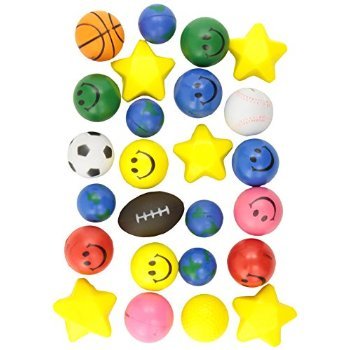The image is a vibrant and playful color photograph featuring a diverse assortment of small, whimsical toys, possibly beads or mini-erasers, laid out in a grid pattern. The collection includes a variety of round objects such as a soccer ball, basketball, baseball, and dodgeball, as well as numerous beads with smiley faces in blue, pink, orange, and green hues. Yellow stars are dispersed among them, eschewing an overall cutesy and cheerful design. The scene is vividly colorful and exudes a joyful ambiance, with every element suggesting it’s a playful assortment intended for children's enjoyment. The overall impression is one of happiness and fun, with a mix of sports-themed items and charming smiley faces all arranged in no particular container, creating a visually appealing and lively image.